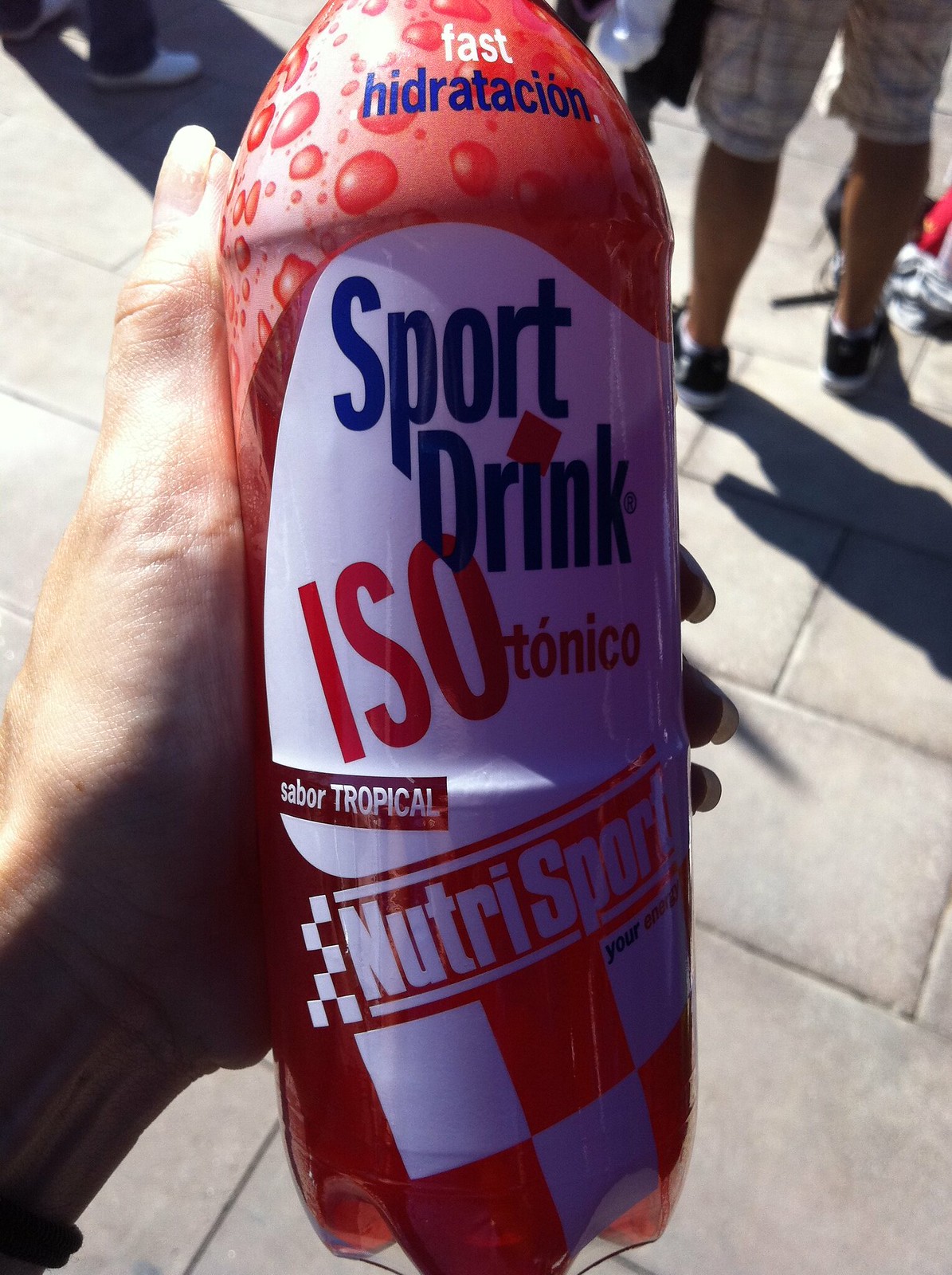A vertical rectangular photograph captures an outdoor scene predominantly featuring a paved walking surface as the background. In the upper right corner, the lower portion of a person is visible, showing only their legs clad in shorts, facing away from the camera. Dominating the lower left part of the image is a hand, palm-up, extending diagonally. The hand holds a large, narrow plastic bottle. The bottle's label features the word "F.A.S.T" in red at the top, followed by "HYDRATION" in blue. The central section of the label showcases "SPORT DRINK" in blue against a white backdrop, with "ISOTONICO" in red below it. The bottom of the label is bordered by a red and white checkerboard pattern.